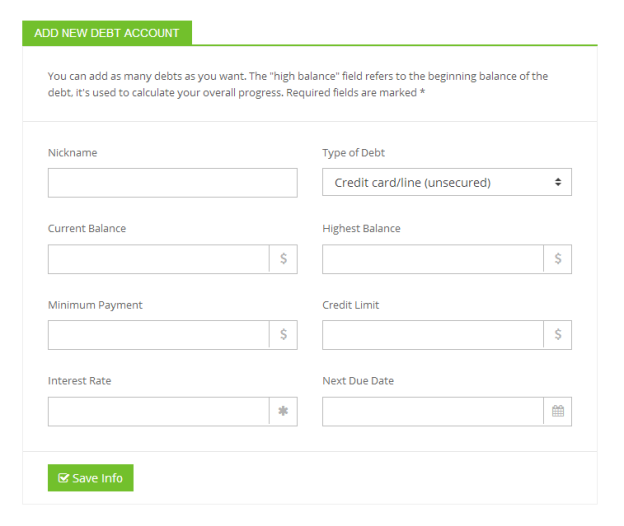**Detailed Caption:**

The image shows a screenshot of a computer interface for adding a new debt account. At the top of the webpage, there's a prominent green bar extending across the entire screen, with a green box attached to it that reads "Add New Debt Account." Just below this, a message informs users that they can add as many debts as they want. The phrase "high balance" is quoted, clarifying that it refers to the initial balance of the debt, which is utilized to calculate overall progress. Required fields are indicated with an asterisk.

As your eyes move down the page, the left side displays empty input fields labeled "Nickname," "Current Balance," "Minimum Payment," and "Interest Rate." The "Current Balance" and "Minimum Payment" fields include dollar signs, while the "Interest Rate" field features a star symbol.

On the right side, from top to bottom, the interface displays a dropdown menu labeled "Type of Debt," which currently shows "Credit Card/Line Unsecured" with up and down arrows for selection. Further down are empty fields for "Highest Balance" and "Credit Limit," both marked with dollar signs. The "Next Due Date" field is accompanied by a calendar icon, indicating the availability of a date picker.

The overall design is clean and functional, aimed at helping users meticulously enter detailed debt information.